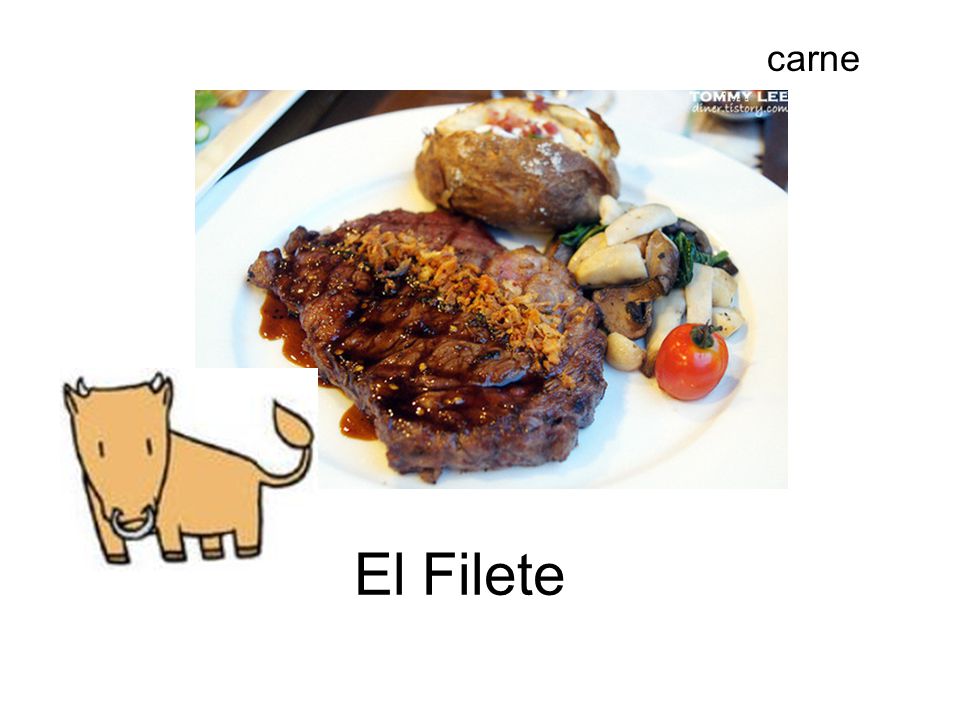This detailed color photograph showcases a meticulously arranged plate of food set on a white plate at a probable dining table. Central to the dish is a thoroughly cooked, well-cut brown steak adorned with brown crumb-like shavings and seasoning. Flanking the steak to its right are cooked mushrooms, a cherry tomato, and slices of a green vegetable. Behind the steak is a baked potato split open and garnished with bacon bits. The photograph includes text: in the upper right corner, "Tommy Lee" and "DinerHistory.com" are displayed in white, while "Carne" is printed in black in another description. A playful, light brown 2D cartoon bull with a nose ring and small white horns appears in the bottom left corner. Below the image, black text reads "El Filete" or "El Filet," hinting at the dish's name. The scene is set on a brown table, with the faint edge of another plate visible in the upper left, adding context to the dining setting.